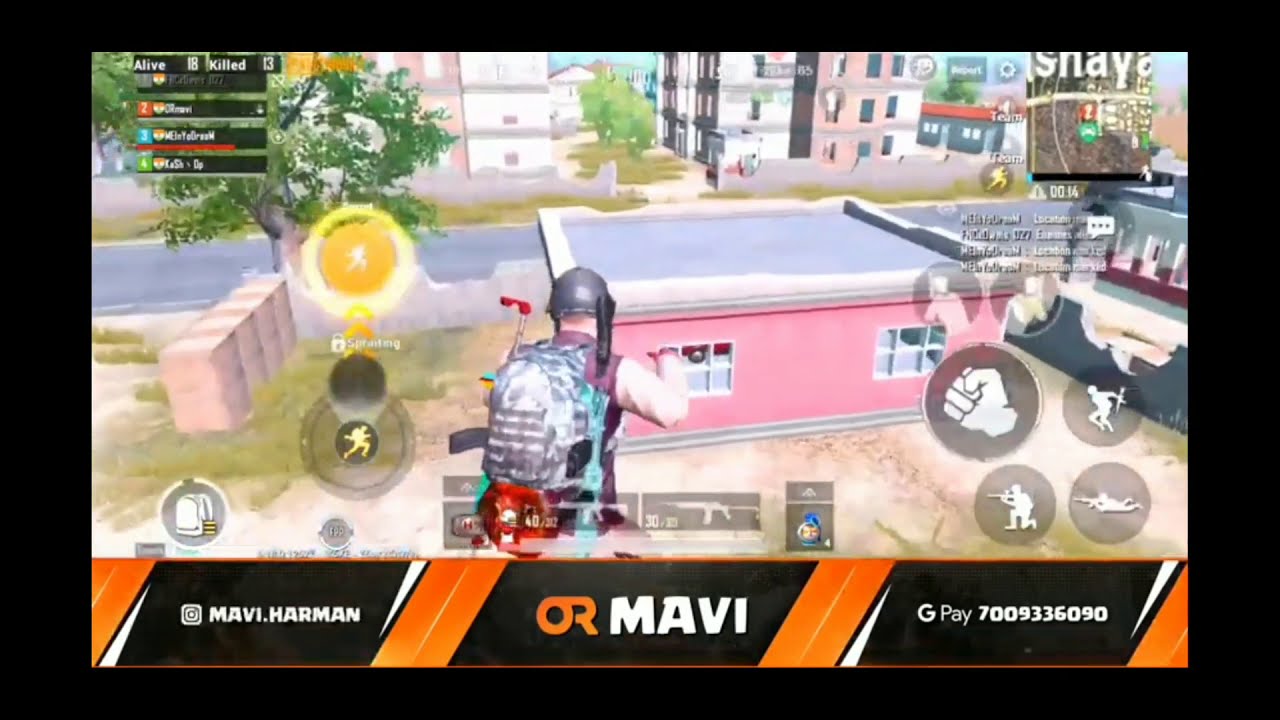In this colorful and dynamic screenshot from a cartoonish video game, a character is depicted mid-jump or levitating in the air. The character, whose back is facing the viewer, is outfitted in a grey helmet, a sleeveless shirt, and an army-style backpack. To the character's left is a gun with a distinctive red handle. The background showcases a small, one-story red building with two windows and a flat grey roof. Beyond this building, a road passes by, lined with taller, multi-story buildings. Added details include trees and patches of grass, along with a secondary character visible across the street.

The game's HUD elements are prominently displayed: symbols including a fist, a man laying down, a man going prone, and others indicating various actions like jumping and shooting. The bottom of the screen is adorned with a black and orange layout containing four brown rectangles separated by an orange section, with the center one marked "ORMAVI," and nearby labels reading "maybe.hearthairman" and "GPAY7009336090." The visual atmosphere is further detailed by a surrounding black outline, making the scene vivid and immersive.